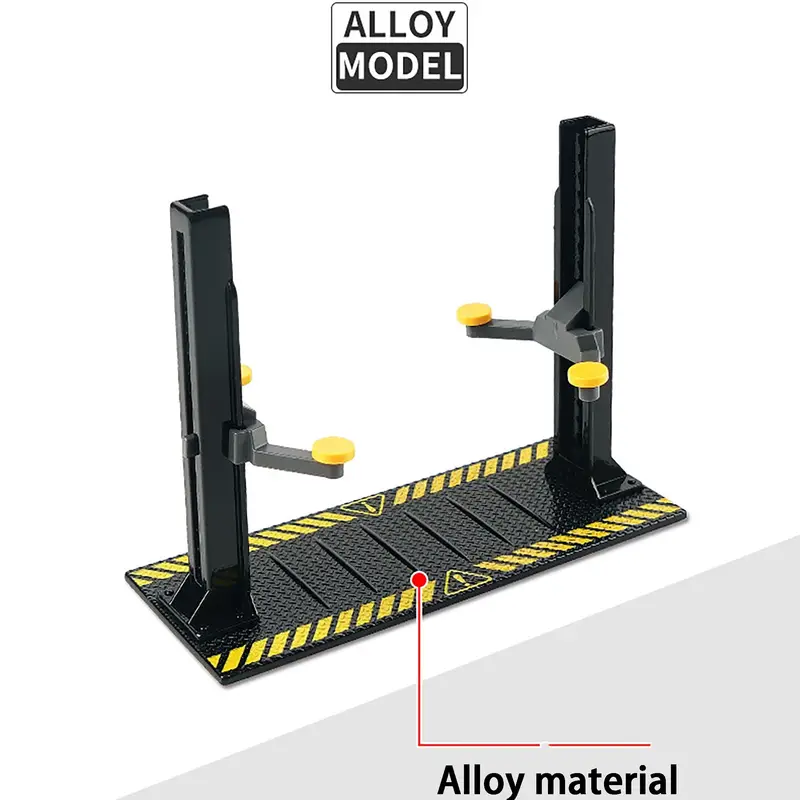The image displays a black metal structure identified as an "alloy model," with instructional text at the top and "alloy material" noted at the bottom. The structure features a rectangular black base with yellow trim along the edges, highlighted by warning symbols in the form of yellow triangles with exclamation marks. Stabilized on this base are two steel beams, each equipped with two arms. These arms end in yellow pads or caps, appearing to function as a clamping or lifting device. The device is shown against a white surface, and there is a large gray triangle taking up most of the right corner, extending to a point on the left. Despite the detailed description, the exact purpose of the device remains unclear.